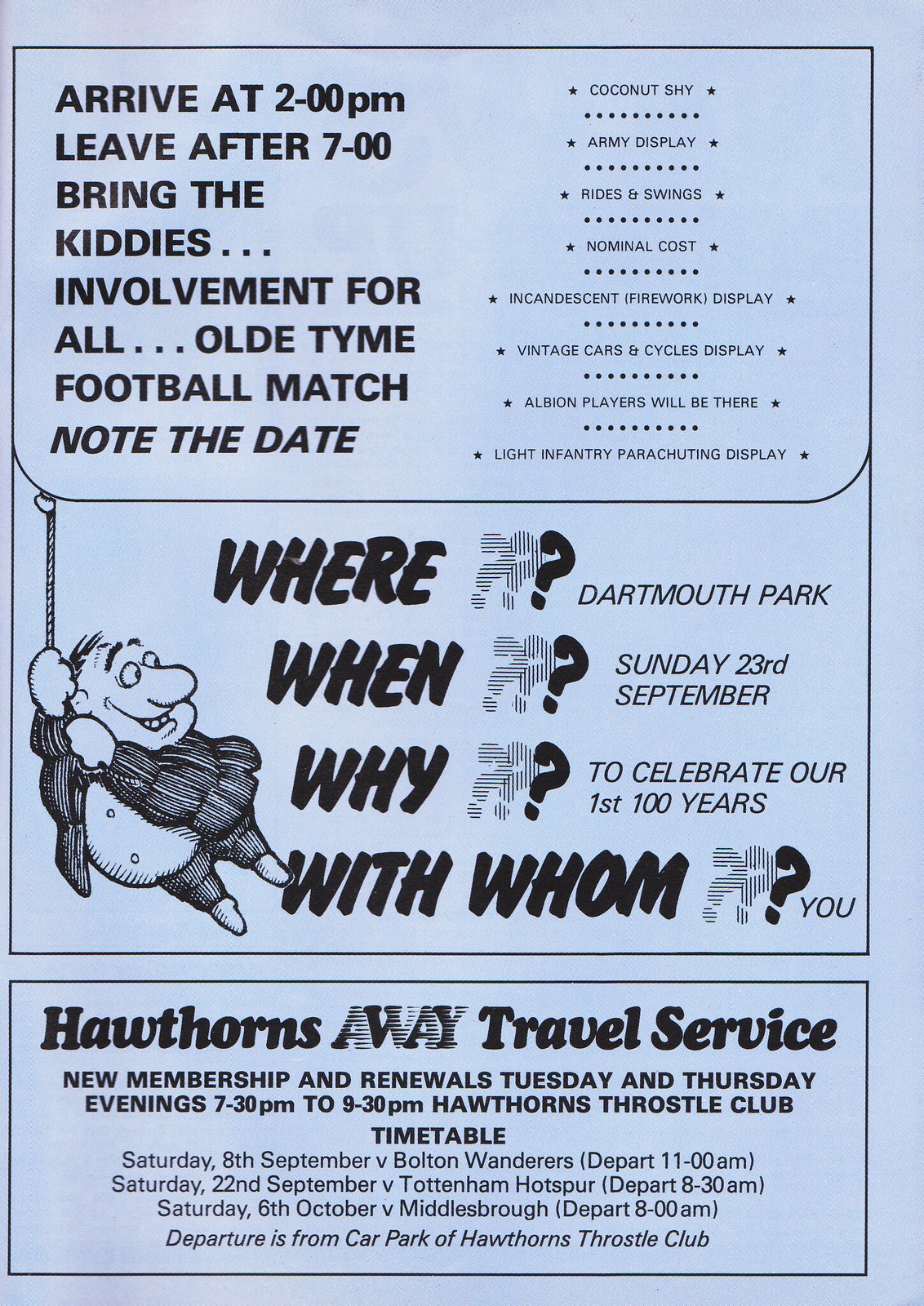The image depicts a black-and-white printed advertisement page from a vintage magazine or football club program, set on light blue paper. It is in portrait orientation, dominated by a rectangular sign bordered in black with various details. The top heading reads: "Arrive at 2 p.m., leave after 7 p.m., bring the kiddies, involvement for all, old-time football match, note the date." To the right, there are bulleted points listing activities such as cost details, fireworks, and car display information. In the middle, there is an illustration of a potbellied man with a large nose, holding a balloon string, looking to the right. The balloon contains text detailing the event specifics: "Where? Dartmouth Park. When? Sunday 23rd September. Why? To celebrate our first 100 years. With whom? You." The bottom section features a horizontal advertisement for "Hawthorne's Away Travel Service," promoting new memberships and renewals on Tuesday and Thursday evenings from 7:30 p.m. to 9:30 p.m., alongside the mention of "Hawthorne's Thoughts of Club." The overall style exudes a charmingly old-fashioned, celebratory tone, highlighting a significant 100-year anniversary event.